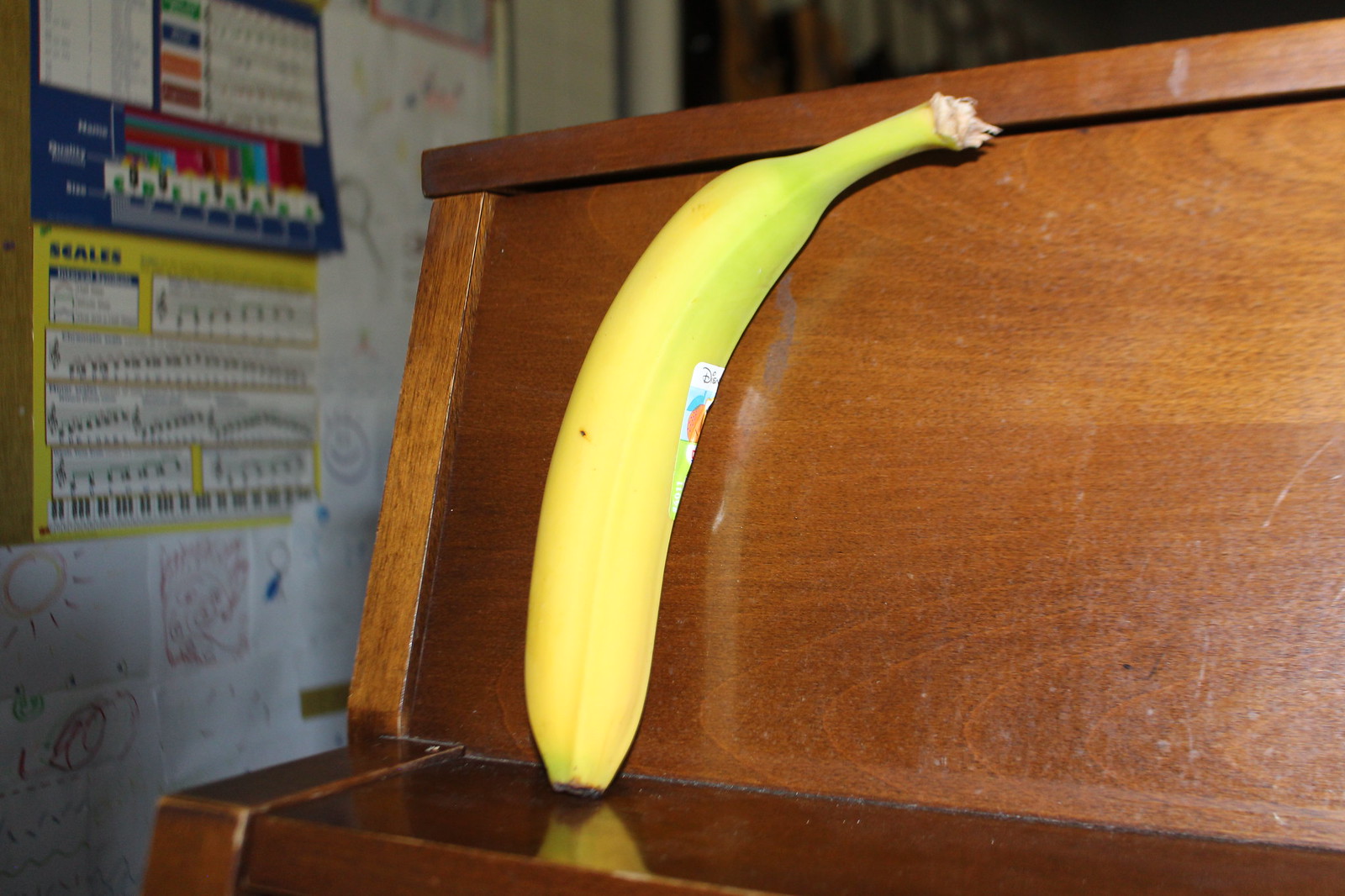The image features a detailed close-up of a meticulously polished wooden countertop with a unique design, showcasing a narrow ledge running alongside its edge. The countertop’s surface is so finely polished that it mirrors the objects placed on it. Centrally featured is a pristine, vibrant yellow banana, almost blemish-free save for a tiny brown spot. The banana’s store label, colorful and intact, is still adhered to its peel. Perched upright on the narrow ledge, the banana's reflection is clearly visible on the lustrous surface of the counter. To the left side of the frame, a wall adorned with various posters and a calendar can be seen, adding a touch of lived-in ambiance to the scene.